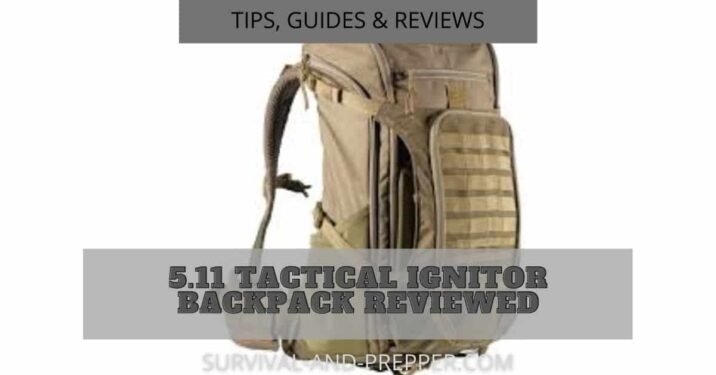This image features the 5.11 Tactical Igniter Backpack prominently centered against a clean, white background. The light brown or tan khaki backpack is detailed with various pockets, zippers, and straps, suggesting extensive storage and functionality. A touch of green can be noticed at the bottom part of the backpack. Positioned such that only one strap is visible, the backpack appears slightly turned sideways and sits in free space without being worn or placed on a surface. At the top of the image, a gray banner with black, all-capital letters reads, "TIPS, GUIDES, AND REVIEWS." At the bottom, another gray banner with darker gray all-capital letters states, "5.11 TACTICAL IGNITER BACKPACK REVIEWED," and just below it, the website "survivalandprepper.com" is displayed in all capital letters in white and gray. This setup suggests that the image is part of an online catalogue or advertisement on a survivalist website, emphasizing the practical and tactical nature of the backpack.